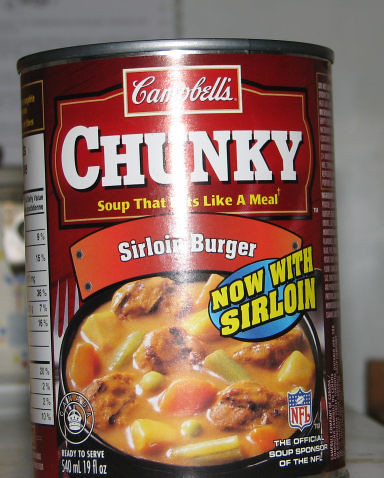In this photograph, the focal point is a single can of Campbell's Chunky soup, occupying approximately 90% of the center frame. The can prominently displays its front label, showcasing the brand name "Campbell's Chunky" alongside its tagline "Soup That Eats Like a Meal." The specific variety, "Sirloin Burger," is highlighted, with an additional blue background emphasizing the words "Now With Sirloin." Below the product name, the label also notes that Campbell's is an official soup sponsor of the NFL and that the soup is ready to serve. The design of the label is predominantly red, featuring white text with selective yellow accents. The background of the image is out of focus, revealing a blurry gray and off-white wall that contrasts softly with the vivid colors of the can's label.